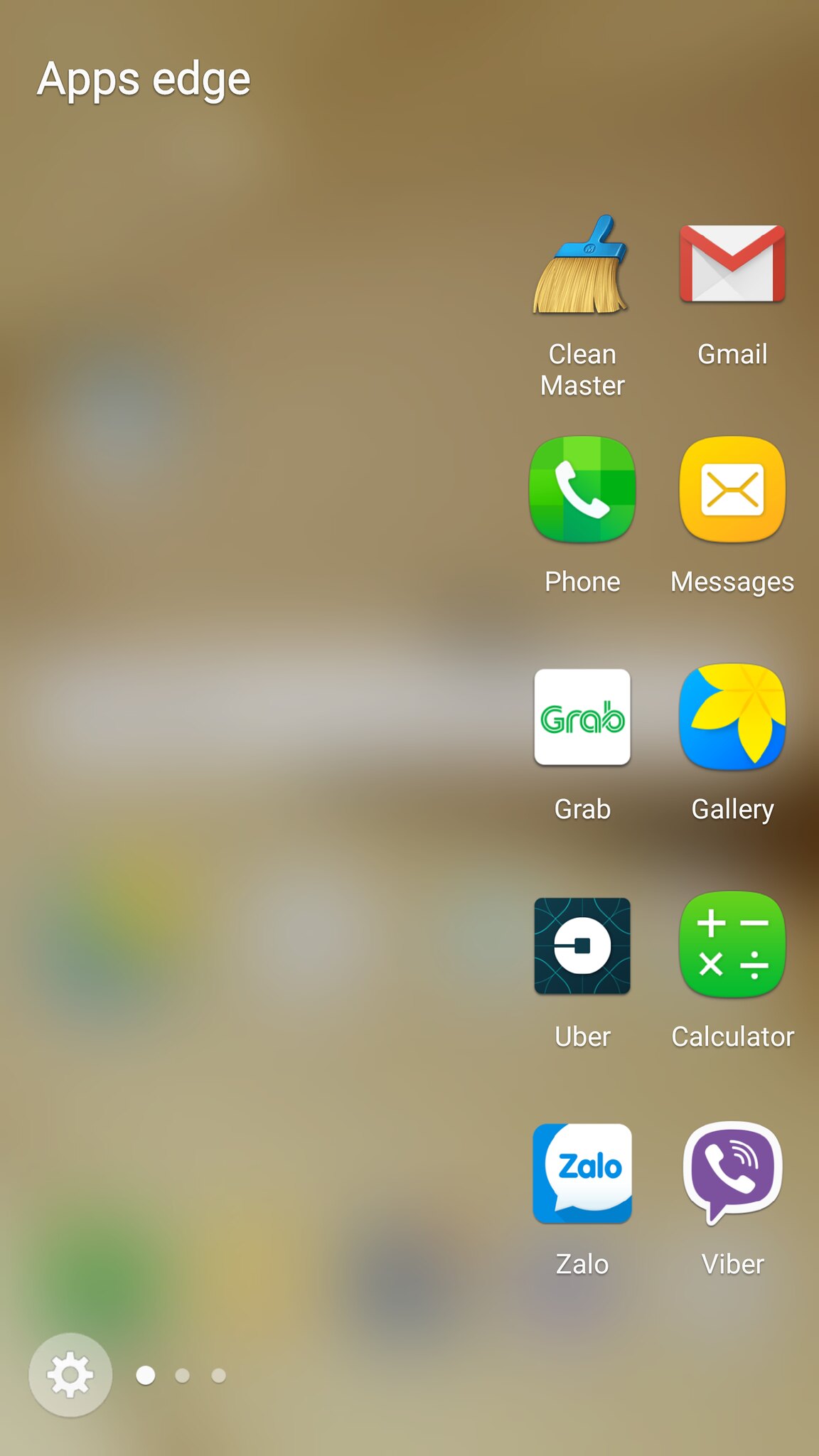This image showcases the home screen of an older Android phone, characterized by a collection of distinct app icons predominantly visible on the right side while the left side remains blurred. The specified icons represent a mix of applications, capturing a snapshot of a more vintage Android user interface. Notably displayed at the top is the classic Gmail app icon featuring a red and white envelope, indicative of a past design. Below it are various other application icons: 

1. **Clean Master** featuring a broom with a blue handle
2. **Phone** marked by the classic green background with a phone symbol
3. **Grab** in green and white
4. **Uber** with its older, more dated logo
5. **Vallo** depicted with a white and blue chat bubble
6. **Gmail** again, identifiable by its red and white envelope
7. **Text Messages** indicated by a yellow background with an envelope design
8. **Gallery** for photos, shown with a blue and yellow icon
9. **Calculator** showcasing standard math symbols on a green background
10. **Viber** represented by a white phone and speaker icon on a purple background

Additionally, the image includes the signature Google search bar, albeit blurred, running horizontally across the screen's midsection. This combination of icons and elements creates an illustrative overview of a bygone Android interface, highlighting a diverse assortment of apps common to older mobile experiences.